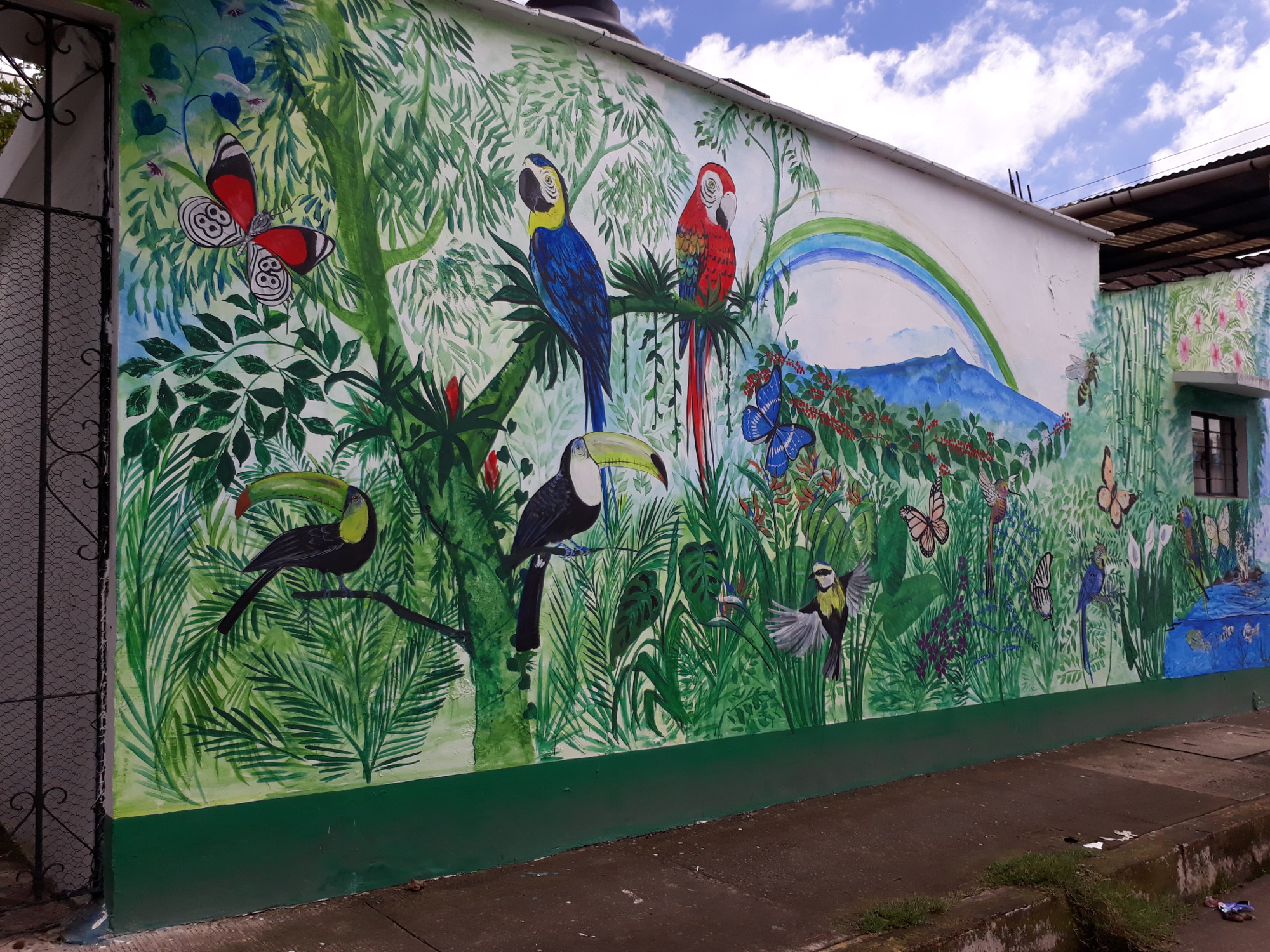The mural, displayed on a white adobe wall outside a building that could be someone's hacienda or a public structure, presents a vibrant tropical scene with a watercolor feel. Dominated by a bright blue sky with fluffy clouds, the mural showcases lush jungle foliage, palm trees, and palm fronds. Prominently featured are various birds: several toucans perched on branches, two large blue and red parrots at the top of a tree, and several different types of butterflies, including a striking blue and a red one. Interspersed among the birds and foliage are delicate pink and green flowers. A distinctive feature is a two-toned rainbow—green and blue—arcing above a distant blue mountain range. Below, glimpses of a wet sidewalk with a little trash suggest recent rain, enhancing the natural and lively atmosphere of this detailed and colorful street art masterpiece.